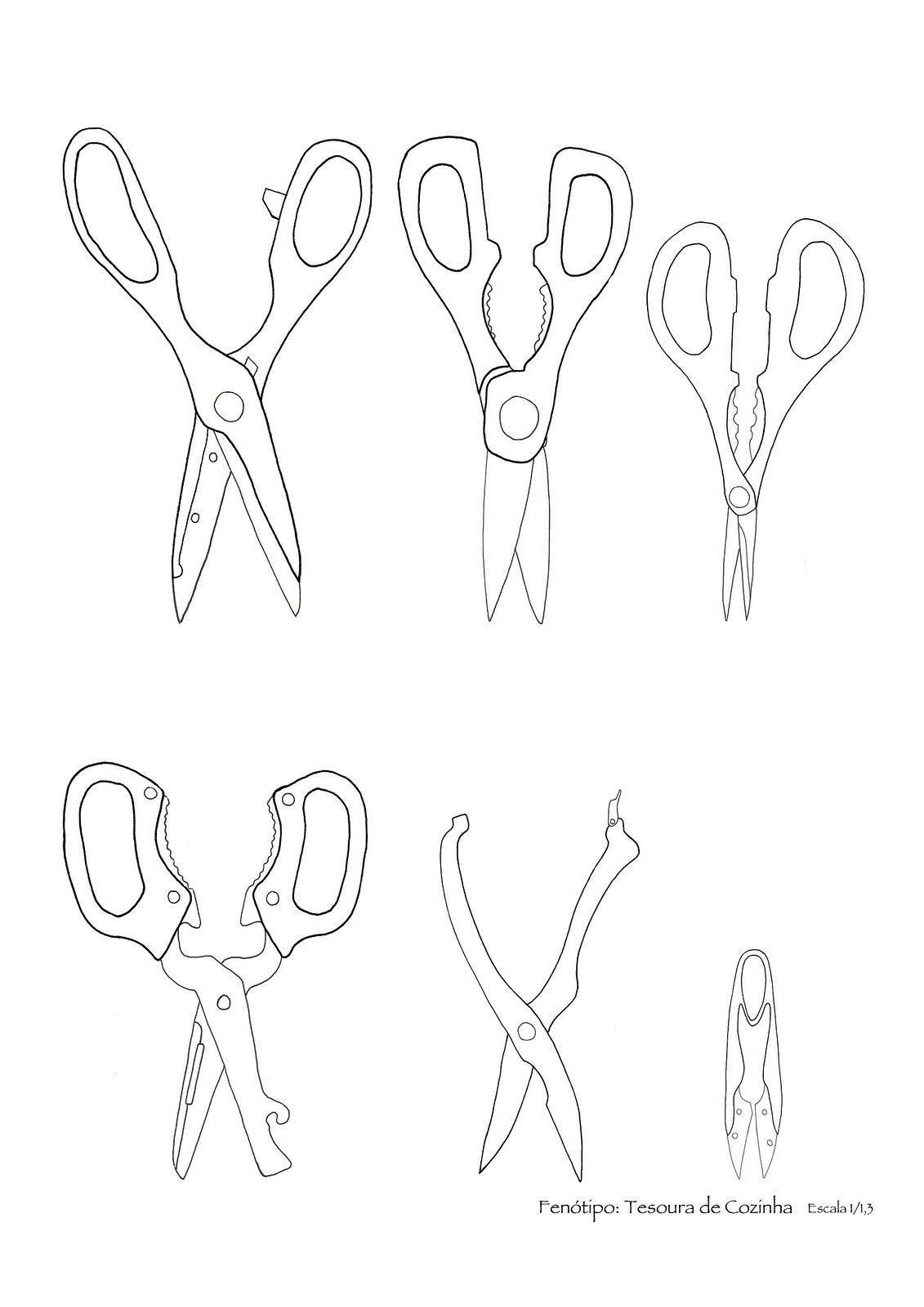This image from a book or magazine features a detailed black and white drawing of six different scissor-like tools arranged in two rows. The top row showcases three distinctive pairs of scissors. The first pair, being the largest, features a clip within the finger loop for securing the blades together. The second pair includes a circular pivot with jagged edges, while the third pair, smaller yet thicker, also has these jagged tensions at the center. The bottom row introduces another array of unique tools. The first tool resembles a bottle opener with one blade ending in a small hook. The second item appears as a cutting instrument devoid of finger loops, akin to tongs or tweezers. The final tool on the bottom row is designed to be squeezed from the exterior, resulting in small, closely-aligned blades. Additionally, there is a depiction of a woman with the artist's unreadable signature near the bottom, adding a personalized touch to the detailed and artful illustrations. No text accompanies the image, emphasizing the artist's intricate renderings of each tool.